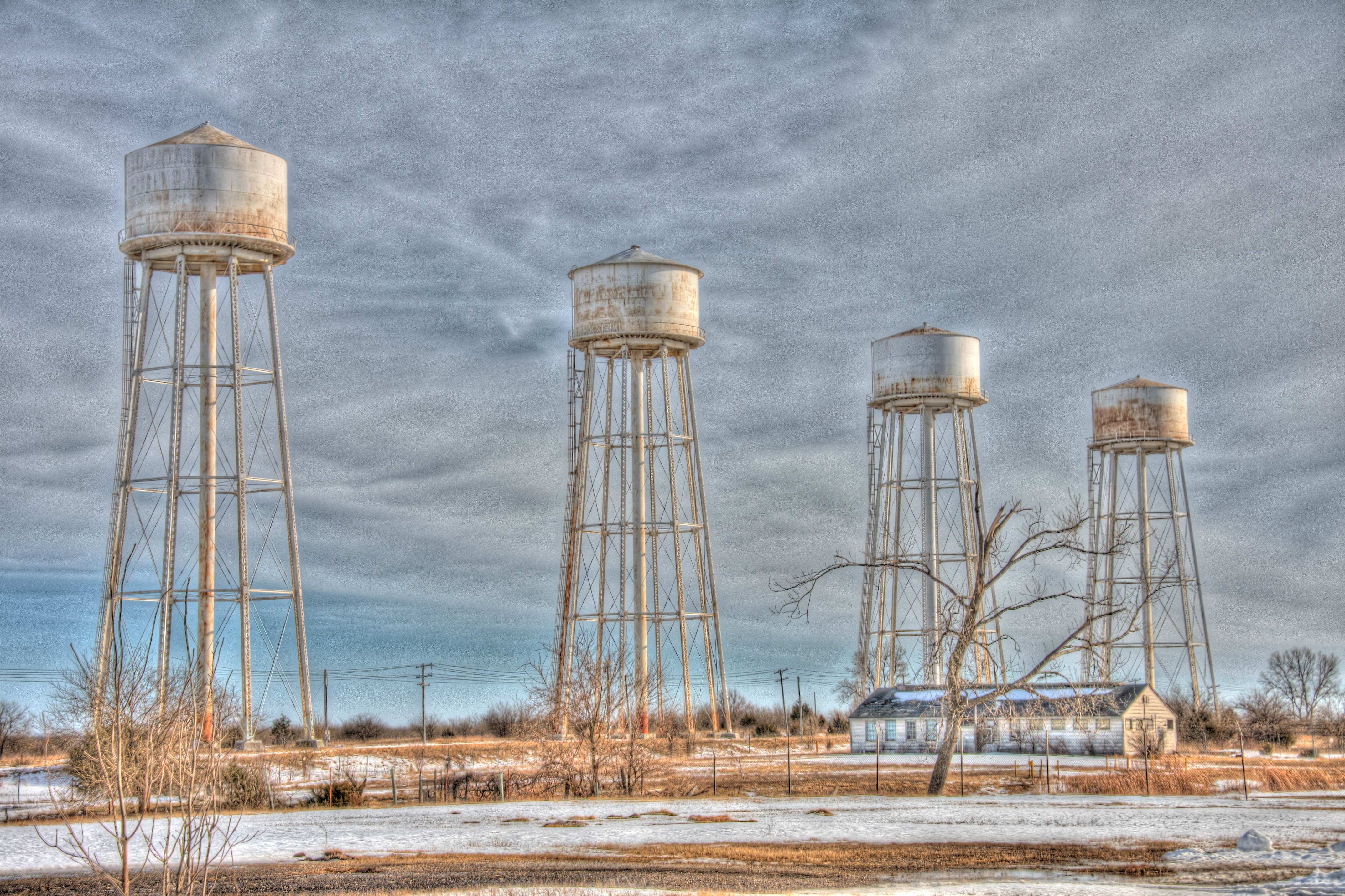The photograph captures an angled view of four tall, rusted, and old water towers, each silvery with a pointed top and lined up in a straight line, many feet apart. The towers are heavily rusted, with the one on the far right showing the most corrosion. The gray, cloudy sky dominates the scene, suggesting cold weather, though a hint of blue is visible near the horizon. In the background, to the right, stands a wide, white one-story house with a black roof layered with snow, surrounded by a fence. The property includes a large, brittle, brown tree, possibly dead or winter-defoliated, and smaller decorative trees, similarly brown and sparse. Dead grass and patches of snow cover the ground in the foreground, and power lines stretch across the horizon.